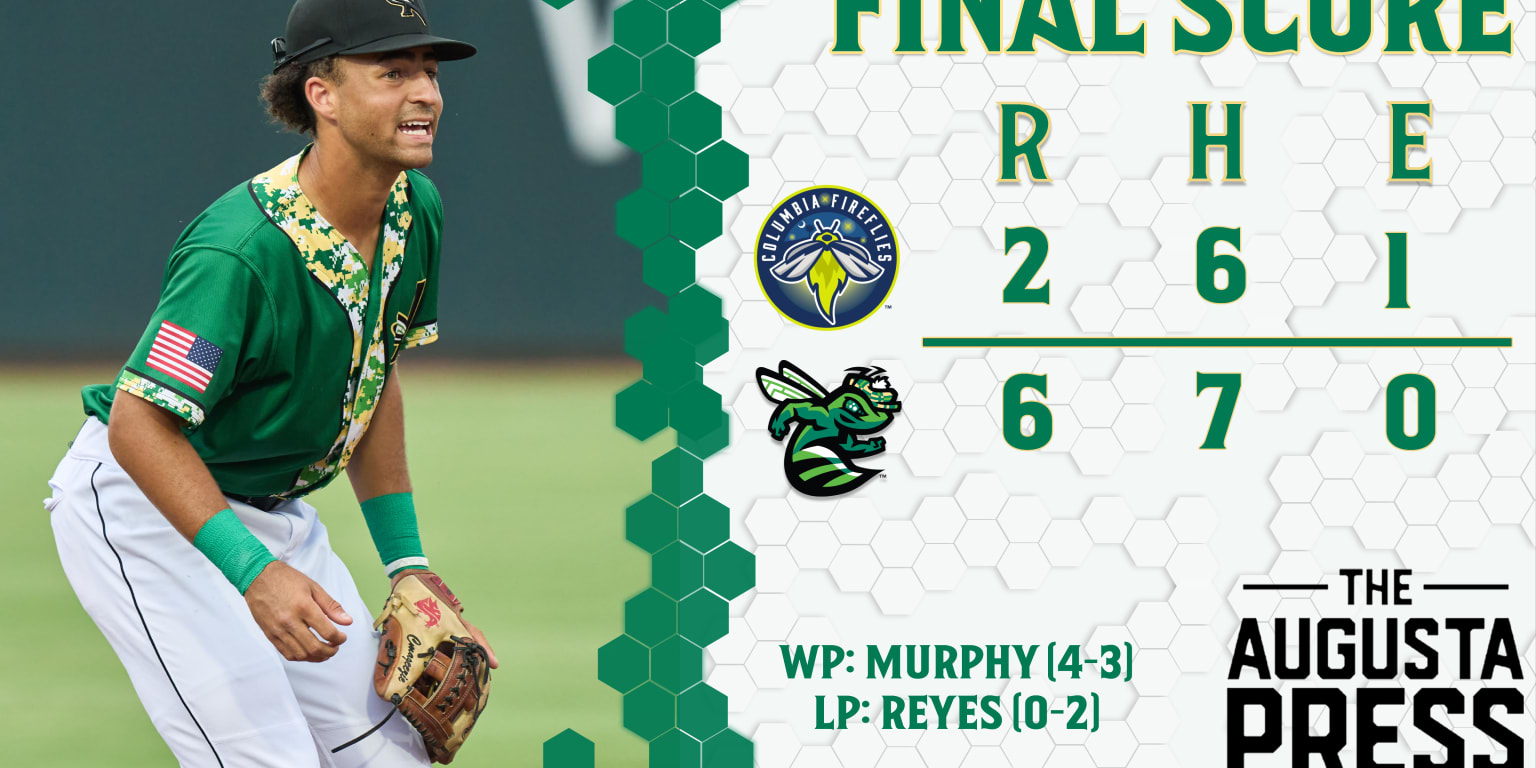In this detailed image, we see a baseball player of likely Latin descent with dark, light brown skin and curly, frizzy hair, captured from what appears to be a graphic or still frame from a sports broadcast. He is facing the right side of the image, wearing a black cap, a green jersey, and white pants that feature black stripes. The collar and the inside of his jersey are decorated with a floral pattern that includes green, yellow, and white colors. An American flag sticker is visible on his right sleeve. His wrists are adorned with green-colored arm guards, and he is holding a mitt in his left hand. The background is blurred, hinting at a stadium setting.

To the right of the player, the final score is displayed: R-H-E stands at 2-6-1 for one team and 6-7-0 for the other. Above this score, an icon of a bee is shown, with a green bee icon at the bottom. The scoreboard text is set against a beehive hexagonal background in green and white, with the text itself in green or black. It says WP Murphy 4-3 and LP Rays 0-2, indicating the winning and losing pitchers. The logos for the teams include representations, one of which is the Columbia Fireflies and the other featuring a green Hornet. This appears to be information from the Augusta Press.